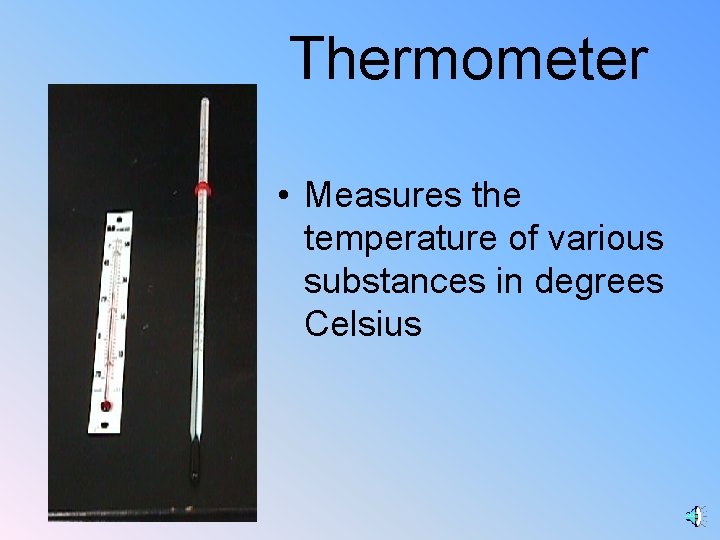This PowerPoint slide features a light blue background that gradually darkens towards the top right and pales towards the bottom left. The slide has a title at the top in black text that reads "Thermometer". To the left, within a vertical black rectangle, there are photographs of two mercury glass thermometers. One thermometer is free-standing with a slim glass tube designed for oral use, while the other is mounted on a flat, white background, possibly part of its packaging. To the right of these images, there is a single bullet point of text that explains: "Measures the temperature of various substances in degrees Celsius." In the bottom right corner, there's a blue and white bullhorn icon, indicating a sound option. The color palette includes shades of blue, black, white, red, and pink, suggesting a clear and straightforward presentation style.